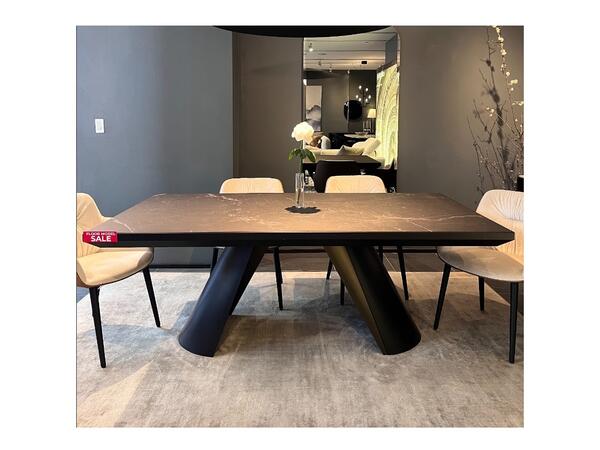This photo showcases a dining table set prominently displayed, likely in a furniture store. The central feature is the black marble-like table, adorned with subtle white veining. Notably, there's a red 'for sale' sign with white font situated on the left edge of the table, denoting a floor model sale. Positioned around the table are four white chairs with black legs, padded with cream-colored cushions. In the center of the table sits a single white rose in a slender glass vase, with vibrant green leaves extending from both sides of the stem. The setting rests on a cream-colored carpet. The backdrop features a large mirror reflecting more of the store, suggesting additional furniture items on display. The overall scene is carefully arranged to enhance visibility and appeal, emphasizing the table and chair set's design and details.